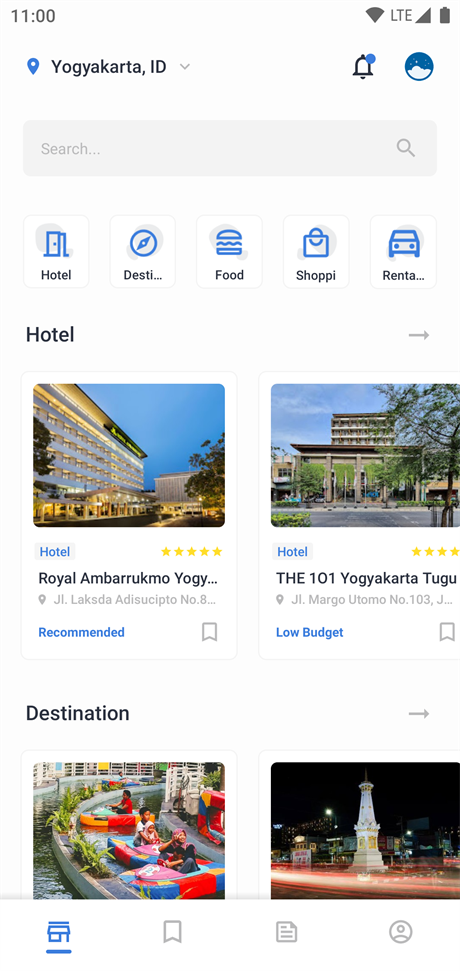This caption describes a screenshot taken from a cell phone, showing the search results for "Yogyakarta, Idaho," with various options for hotels, destinations, food, shops, and rentals. The top of the screen displays the time as 11 o'clock, with an LTE signal and a fully charged battery icon. Below the search bar, there are clickable icons for hotel, destination, food, shop, and rentals.

In the hotel section, two listings are visible. The first hotel is partially named "Royal Ambarakumo Yogi..." and is rated five stars. The second hotel, a budget-friendly option, is named "The 101 Yogyakarta Tegu" and has a four-star rating.

For destinations, the screenshot features images of an amusement park and a cityscape, suggesting potential places to visit in the area.